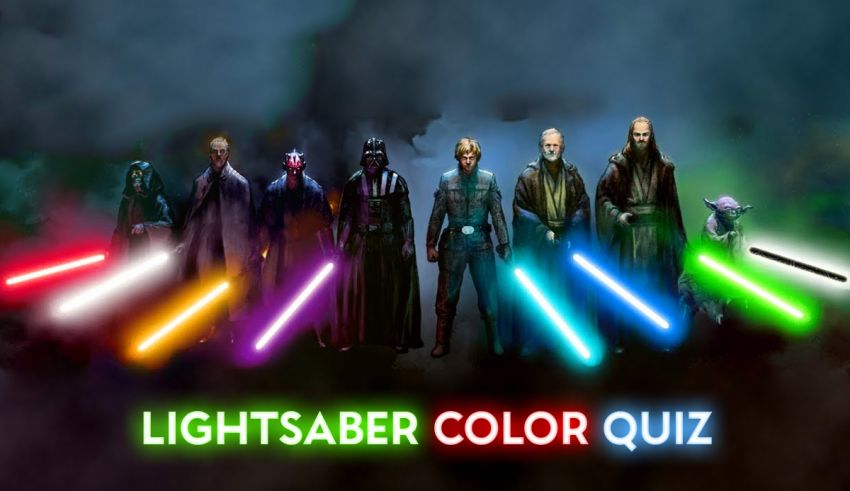This detailed illustration features eight fantasy characters from the Star Wars franchise, standing in a line against a dark background with blue-black clouds, which makes them pop. Each character wields a unique lightsaber with various colors: red, white, yellow, purple, turquoise, blue, green, and black. Notable characters include Yoda, standing on the right with a green lightsaber, and Darth Vader on the left. The middle features a mix of characters, including two men in Jedi costumes. The phrase "lightsaber color quiz" is prominently displayed at the bottom in a multi-color, neon light font: "lightsaber" in green, "color" in red, and "quiz" in blue, adding a vibrant touch to the dark scene.